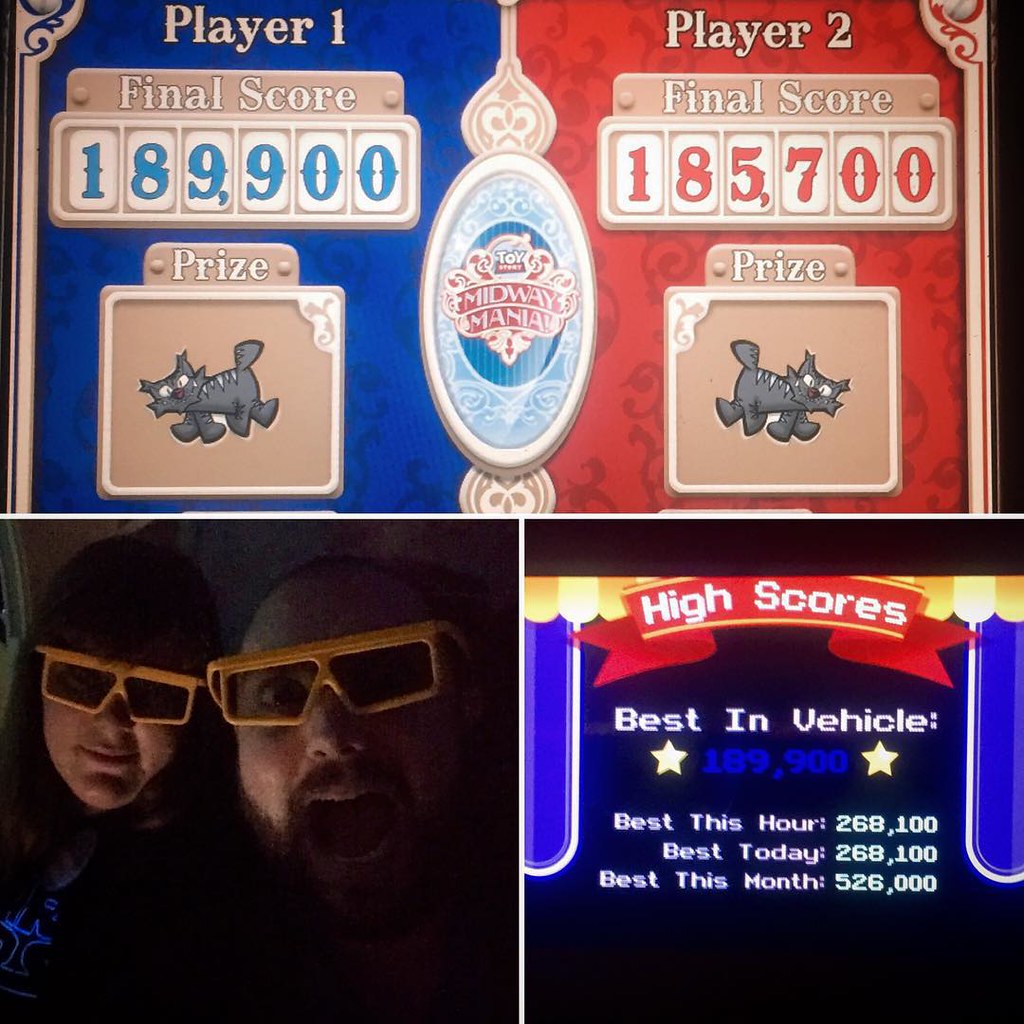The image is divided into three sections, giving it an organized and colorful appearance. The top section features a game interface that depicts a Toy Story-themed carnival game called "Toy Story Midway Mania." The left side displays a blue background labeled "Player 1" with a final score of 189,900 and an image of a fluffy plush toy cat as the prize. On the right side, a red background labeled "Player 2" shows a final score of 185,700 with a similar plush toy cat prize. In the center of this section is a brooch-like graphic bearing the game's title, further emphasizing the carnival theme.

The bottom left section includes a photo of a man and a woman, possibly a couple, seated in a dark environment. The man has a beard, mustache, and is somewhat balding, while the woman has long hair. Both are wearing 3D glasses and are likely at a theme park. The man has his mouth open in excitement, adding to the playful and whimsical atmosphere.

In the bottom right section, a "High Scores" leaderboard is displayed on a black background with a red banner. It shows "Best in Vehicle" at 189,900, "Best This Hour" at 268,000, among other top scores. The varied colors, ranging from blue to red backgrounds and blue to white text, tie together the theme of a competitive yet fun carnival-like experience in a theme park setting.